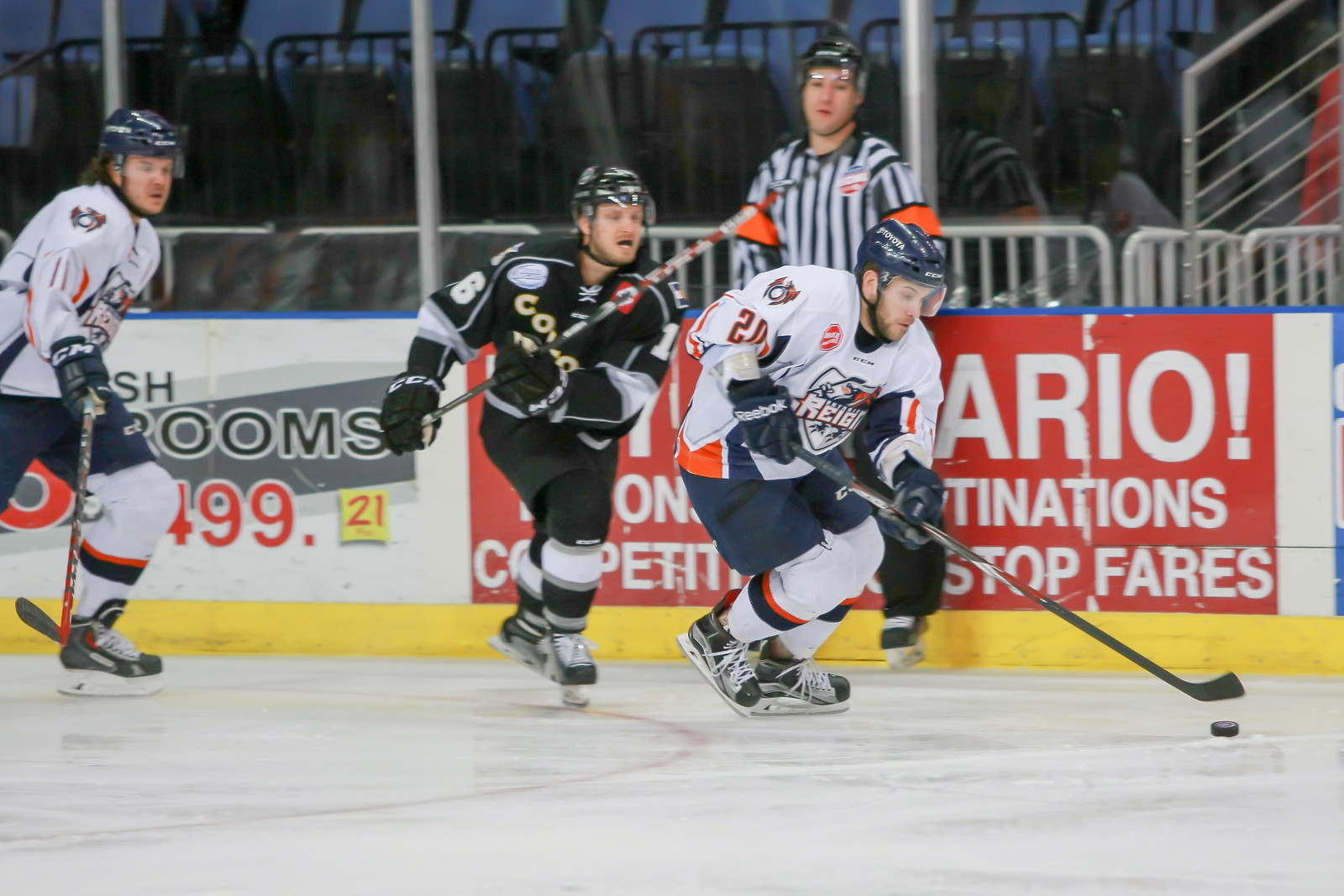In this image, we see a dynamic scene of a hockey match featuring three players and a referee on an ice rink. The referee, identifiable by his black and white striped uniform and helmet, stands behind the players, close to a reflective wall that obscures the full view of the advertisements behind it. The legible part of the writing spells out "fairs" prominently. The player's uniforms are distinct, with two athletes in white jerseys featuring navy shorts, white socks, and orange and navy stripes, indicating they are from the same team. The emblem on their chests appears to say "rain." The player on the right, with the number 20 on his sleeve, is poised with a hockey puck in front of his stick. In contrast, the middle player dons a black jersey with the number 6 on his sleeve, belonging to the opposing team. Behind the players, the half wall showcasing ads partially peeks through, with visible text like "rooms" and "499" in black and red. Meanwhile, another ad in red background reads partially as "A-R-I-O exclamation mark stop fares." The scene captures an intense moment in the game, precisely reflecting the action and distinctive elements visible on the rink.